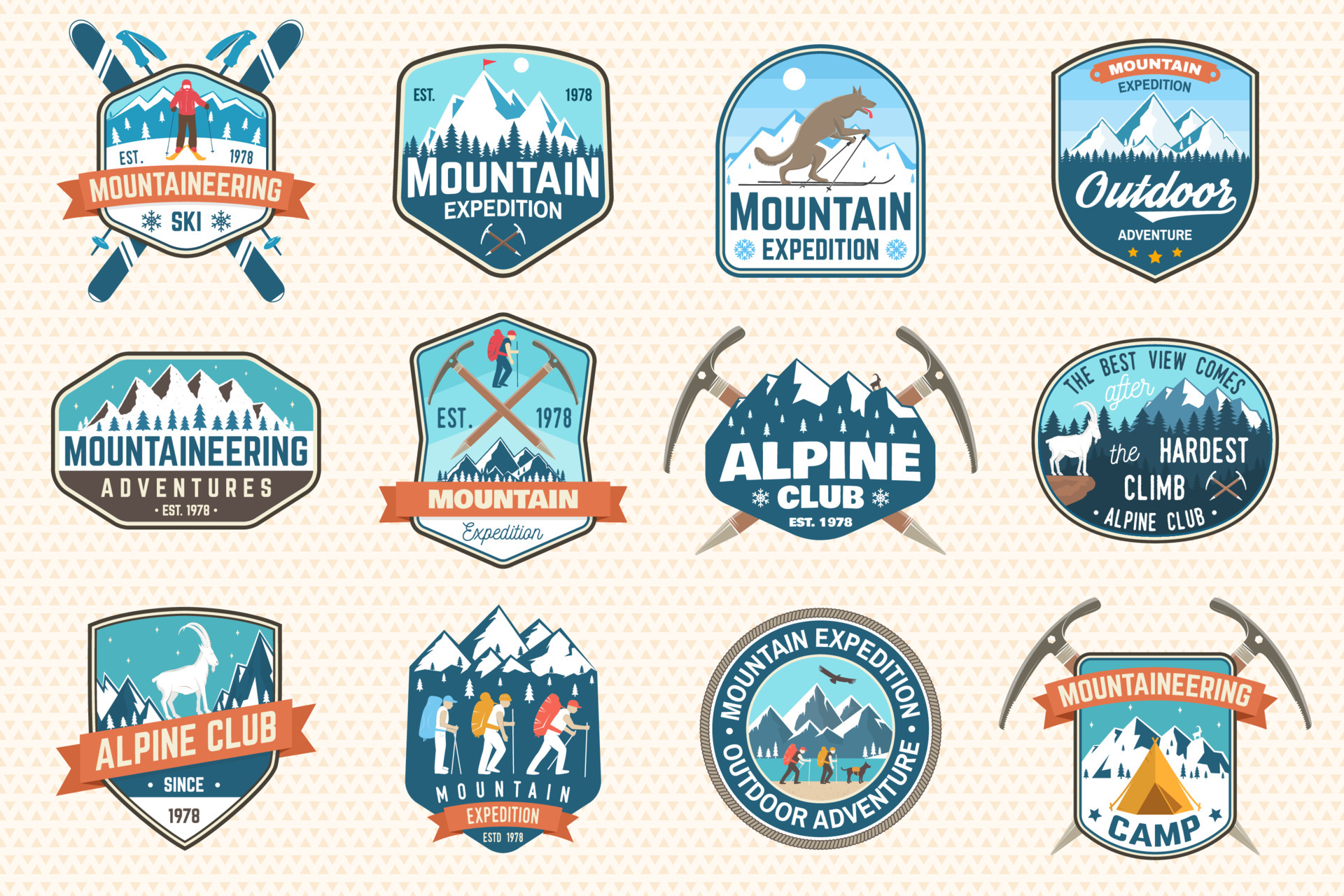The image features a series of twelve company logos on a white and pink background, arranged in three rows with four logos each. Each logo shares a mountain expedition or outdoor adventure theme with dominant colors of blue, white, and occasional touches of orange and brown. 

In the top row, the first patch showcases the word "Mountaineering" on an orange band over a blue and white design. The second is also blue and white, labeled "Mountain Expedition" with a mountain illustration. Next, there is another "Mountain Expedition" logo with a wolf on skis. The last in this row displays "Outdoor" in blue and white, with mountains in the background and "Mountain Expedition" on an orange band.

The second row begins with a "Mountaineering Adventures" patch in blue, white, and brown. Beside it, another patch reads "Mountain" on an orange band with pickaxes crossed at the bottom. The third logo says "Alpine Club," featuring mountains and pickaxes crossing behind the patch, colored in blue and white. The final patch in this row, "Harvest Club," includes mountains and a deer or antelope emblem.

In the bottom row, the first logo shows "Alpine Club" with an orange band on a blue and white patch, depicting mountains and an animal. Next is a patch with mountain tops at the top, three climbers in the middle, and "Mountain Expedition" on an orange band at the bottom. Following that, a circular patch reads "Mountain Expedition, Outdoor Adventure" around the edges with a central mountain image. The last logo presents "Mountaineering" on an orange band, featuring an illustration of mountains, a tent, and the word "Camp," with crossed pickaxes extending from the bottom corners.

The overall design of these patches emphasizes elements of mountaineering and outdoor adventures with prominent images of mountains, skiing, climbers, and nature, unified by a consistent color palette of light and dark blues, whites, and accents of orange and brown.